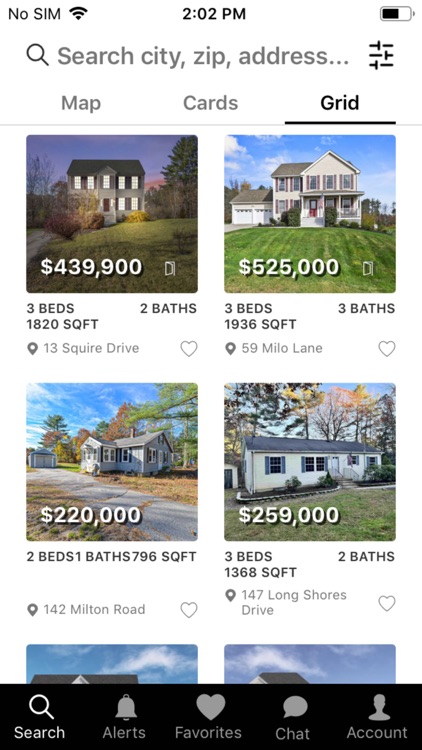This image is a detailed screenshot taken from an iPhone displaying a house-hunting app interface. In the top left corner of the screenshot, there is a 'No SIM' indicator, signaling that the phone lacks a SIM card but is connected to a Wi-Fi network, as indicated by the Wi-Fi icon. The time is displayed centrally at 2:02 p.m., and the battery level is visible on the far right side of the status bar.

The main app interface features a search bar positioned below the status bar, characterized by a magnifying glass icon on the left, followed by placeholder text reading "Search city, zip, address...". Next to the search bar, on the right, is a black filter button, enabling users to refine their search criteria by various factors such as house type, location, and features.

Directly beneath the search bar is a segmented control with three tabs labeled 'Map', 'Cards', and 'Grid', with the 'Grid' tab currently selected. The 'Grid' view displays properties in a two-by-two layout, showcasing various houses side by side. Each property listing includes a thumbnail image of the house, with diverse styles ranging from single-story to multi-story houses and varying exterior colors like white and brown.

Overlaying each house image is the property's price, while additional details such as the number of bedrooms, square footage, and location are listed directly below each image. Each listing also features a heart icon located at the bottom-right corner, allowing users to favorite the property for future reference.